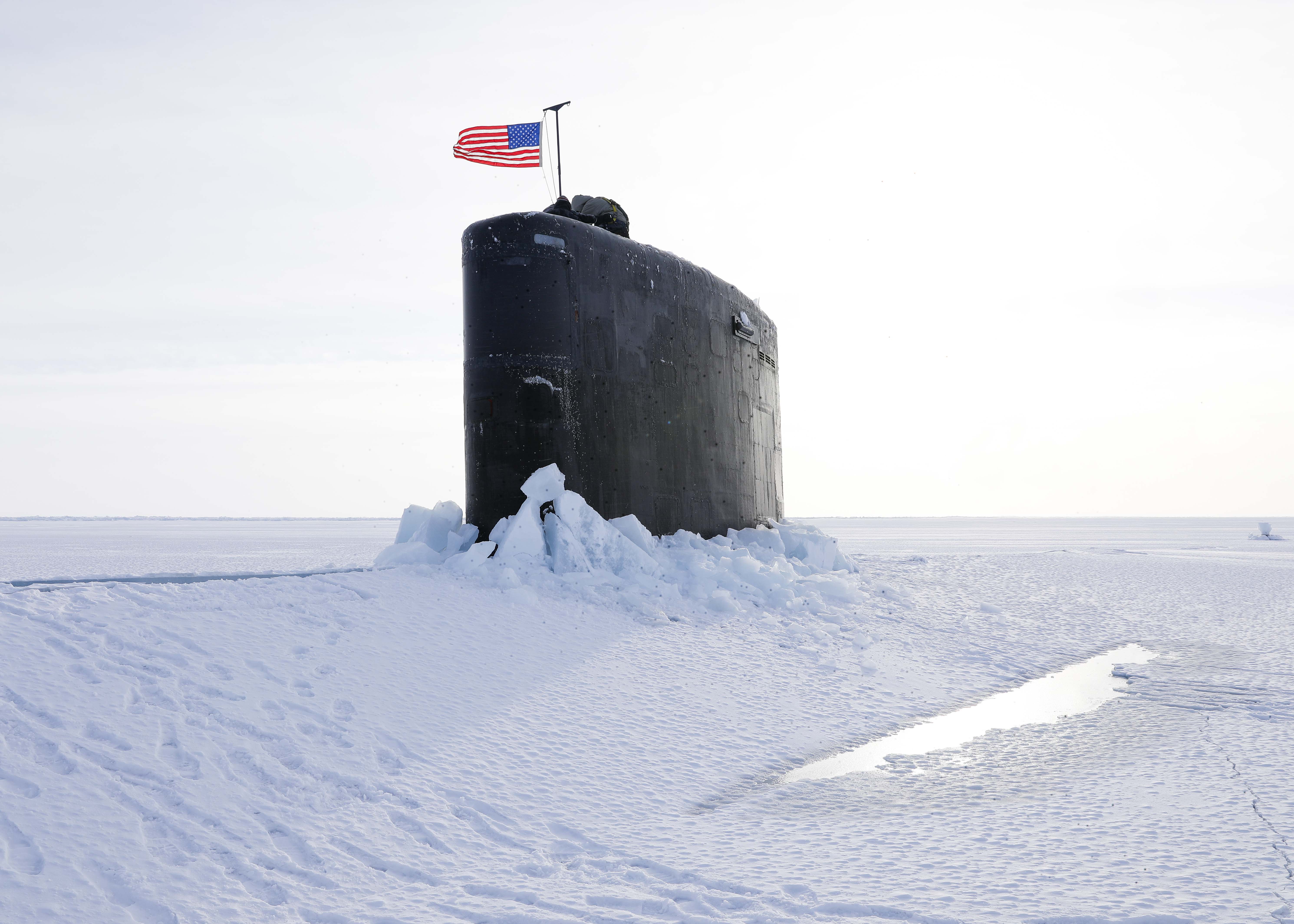This is a horizontal color photograph capturing a stark winter landscape, completely covered in snow and ice. Dominating the middle portion of the image, a black, cylindrical part of a ship, likely a submarine, juts out of the frozen ground. Perched atop this metallic structure is a flagpole proudly displaying the waving United States flag, its red, white, and blue stars and stripes standing out vividly against the monochromatic scene. The background consists of a seamless, white sky, blending with the snow below, creating an almost ethereal effect, particularly on the right side where the whiteness appears even more intense. In the lower right-hand corner, a small water puddle disrupts the otherwise unbroken expanse of snow and ice, its shape stretching from top to bottom. This serene and desolate scene evokes a sense of isolation and tranquility.